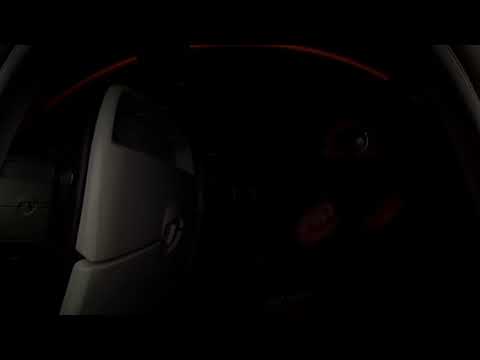This is a very dark rectangular image, likely taken in low lighting or at night. On the left side of the image, there appears to be a gray plastic object, which resembles the back of a car seat or perhaps a door panel, potentially from an airplane. This object seems to be split into an upper and lower part, with the top part possibly functioning as a headrest. In the upper part of the image, there is a red-colored arched line along with several red circular objects that are difficult to identify. Additionally, there are some gray-colored pipes located in the top left and top right corners of the image. The center of the image is mostly solid black, making it challenging to discern further details.